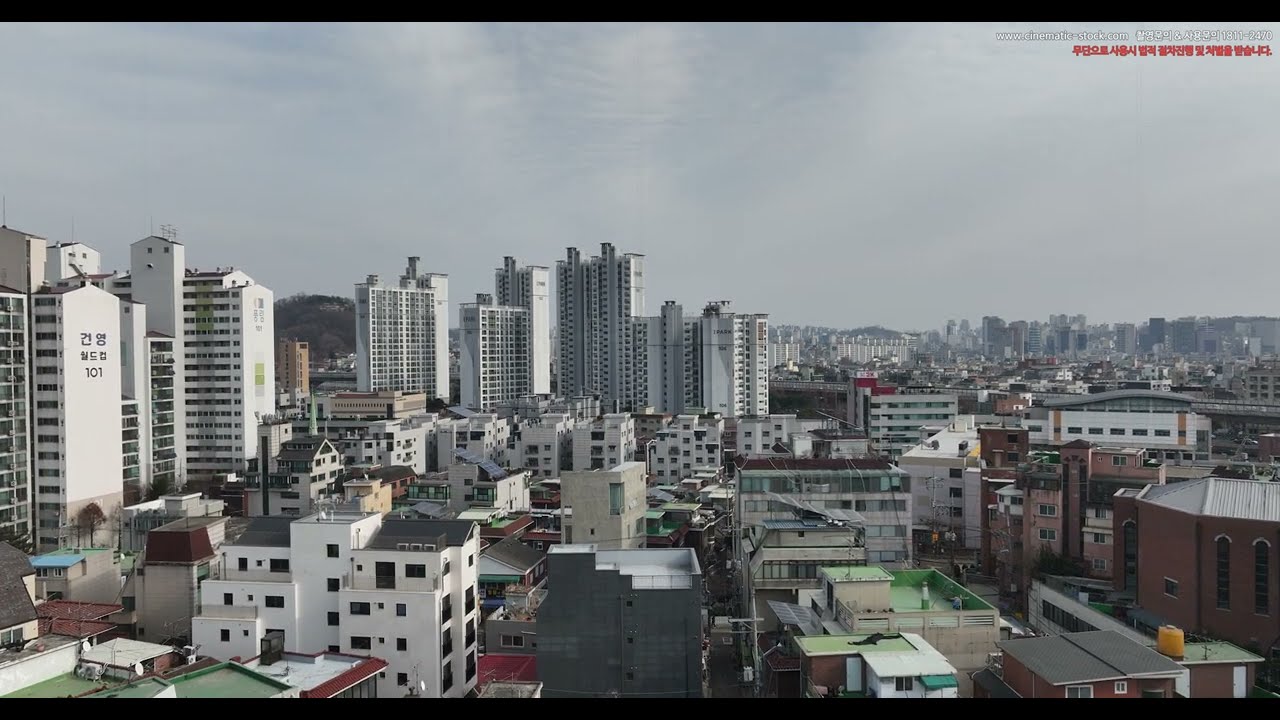The image captures a dense urban cityscape on an overcast day, taken from a high vantage point, possibly atop an apartment building or hotel. The view spans from the foreground to the horizon, showcasing an array of buildings cluttered throughout the scene. Foreground structures vary in height, from lower apartment buildings with red and white facades to taller hotel-like buildings reaching up to 25 stories. Prominent in the left-center, a building featuring Asian script, likely Korean, hints that this is not a U.S. city. The center of the image highlights tall skyscrapers filled with windows, while multiple white and red buildings with balconies and green roofing punctuate the middle and lower grounds. Skyscrapers in the background suggest a bustling downtown area beyond this expanse of tightly packed urban architecture.